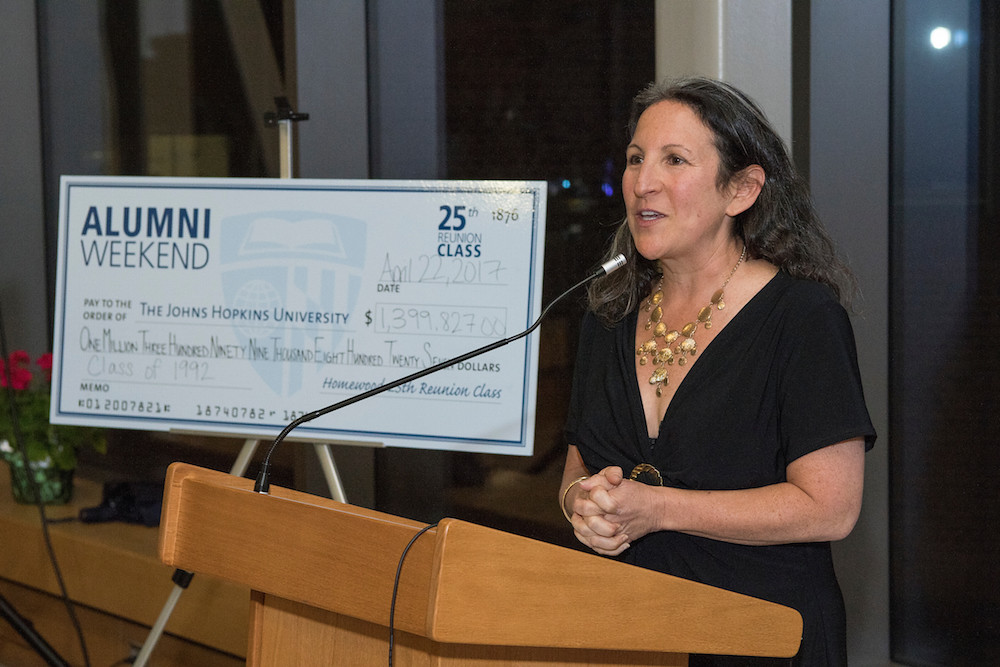In the image, a woman with longish black hair, dressed elegantly in a black dress and wearing a gold necklace with dangly elements, stands behind a wooden podium. A microphone extends toward her face, and her hands are clasped in front of her as she speaks. To her right, there's a tripod stand displaying a giant laminated check. The check details include "Alumni Weekend" in the upper left corner and "25th Reunion Class" in the upper right, dated April 22, 2017. The check is made payable to "Johns Hopkins University" for the amount of $1,399,827.00 and is signed by the class of 1992. The setting appears to be indoors, with a plain background of wall or window coverings, and while the audience isn't visible, it’s clear she is addressing them about this significant donation.